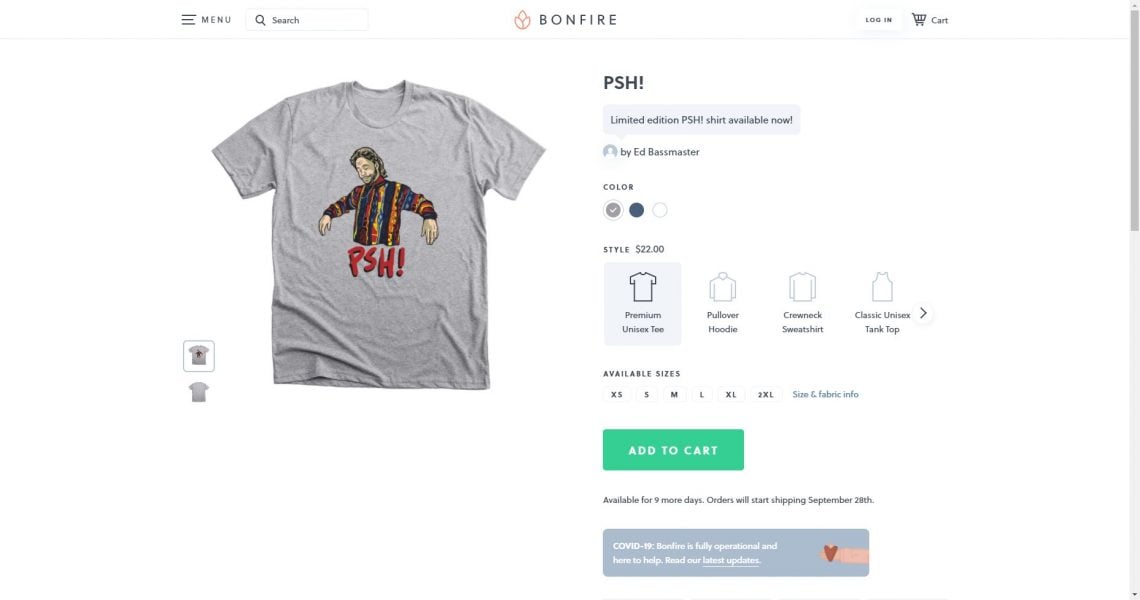The image features a promotional graphic for a limited edition P.S.H. shirt. At the center of the graphic, there's a picture of a man wearing a multi-colored sweater with a distinct, stitched pattern on it. Overlaid on the sweater is a faint display of a light gray shirt showcasing the letters "P.S.H." prominently.

Above the man's image, there is a navigation bar displaying options such as "bonfire," a menu icon (often represented by three horizontal lines), a search bar with a magnifying glass icon, a shopping cart icon, and a login option. 

In the middle of the image, the text "Limited Edition P.S.H. Shirt Available Now" is prominently displayed. Below this text, there is a blank profile picture within a circle labeled with the name "Ed Bassmaster." 

To the side, there are color selection options for the shirt, highlighted in gray, blue, and white, with gray being the currently selected color.